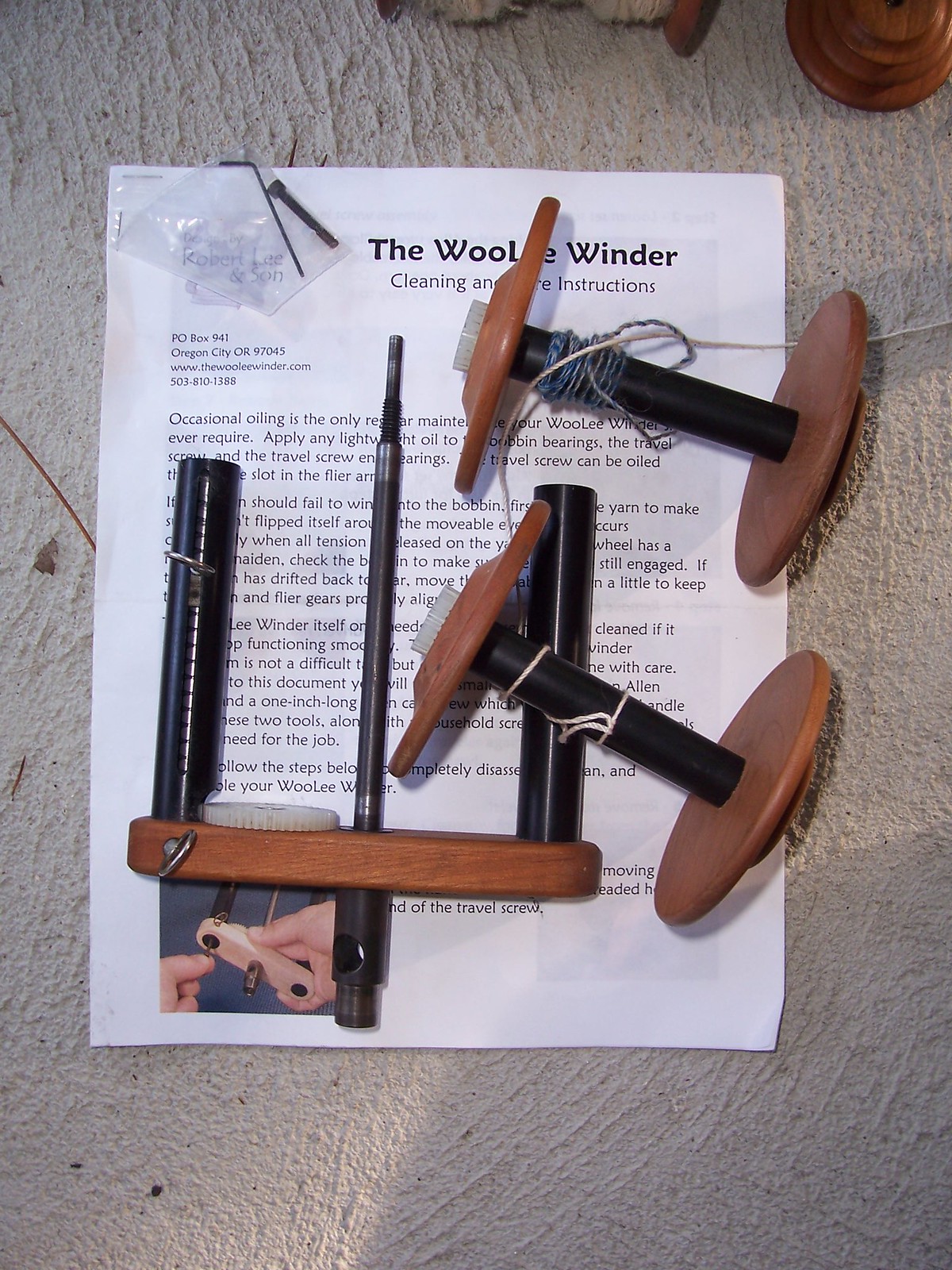This photograph captures a detailed scene of items intended for wool winding, placed on what appears to be a gray concrete surface. The central items are three distinct spindles or spools, each possessing a unique structure. Two of these spools feature a reddish-brown wooden ends and black central cylindrical sections, evident that only a scant amount of thread remains on them. Alongside these, there's a more complex tool situated in the middle, characterized by a long metal rod running through its center, flanked by a flat, oval-shaped wooden component with two vertical black pipes extending approximately six to eight inches, likely designed to accommodate the spools.

Beneath these components, there's a white sheet of paper with partially visible text, headlined as "The Wooly Winder Cleaning and Care Instructions." The paper possibly contains detailed guidance on maintaining and assembling the wool winding apparatus, along with a small colored illustration in the bottom left corner, depicting how the pieces fit together.